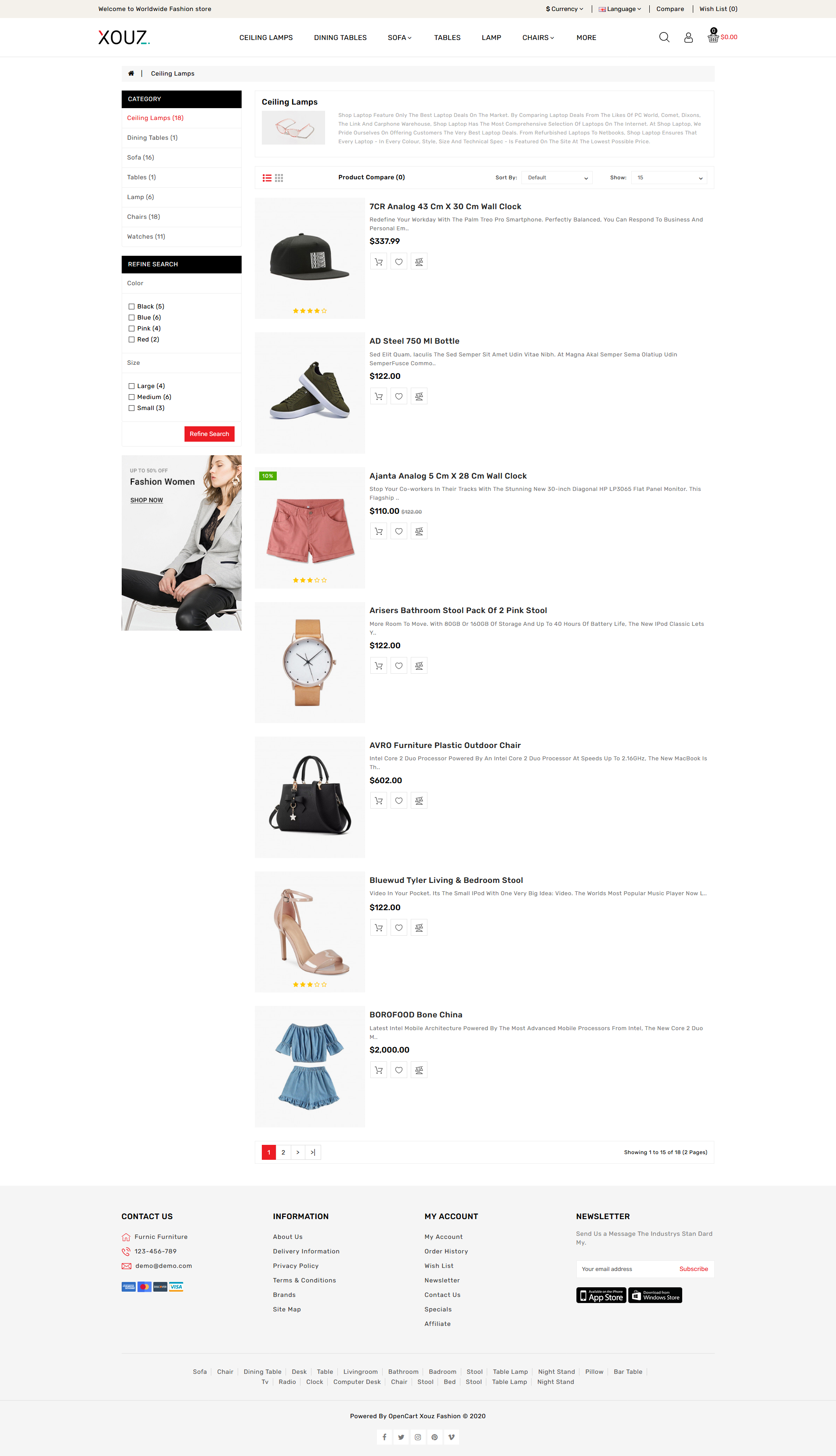**Screenshot of a Fashion and Home Decor E-Commerce Website** 

This image appears to be a screenshot of an e-commerce website focused on fashion and home decor. The interface features a very thin, greyish bar at the top displaying the text "Welcome to Worldwide Fashion Store." To the right of this message, there are options for selecting currency and language, along with links for comparing items and a wishlist.

Below this bar, a navigation menu presents categories such as Ceiling Lamps, Dining Tables, Sofas, Tables, Lamps, Chairs, and more. The shopping cart icon indicates a total of $0.00.

On the left-hand side, there is a vertical sidebar. Currently selected in red is the "Ceiling Lamps" category, which shows 18 items. Additional category options are: 
- Dining Tables (1)
- Sofas (16)
- Tables (1)
- Lamps (6)
- Chairs (18)
- Watches (11)

Beneath the categories is a black box labeled "Refine Search" in white text. This section offers several filtering options:
- **Color:** Black (5), Blue (6), Pink (4), Red (2)
- **Size:** Large (4), Medium (6), Small (3)

A red "Refine Search" button is included to apply these filters.

The main section displays a vertical list of items for sale. Each item is detailed with a product name, description, and specifications. Some of the items listed are:
1. **7 CR Analog Wall Clock**: 43 cm x 30 cm
2. **80 Steel 750 ml Bottle**
3. **Janta Analog Wall Clock**: 5 cm x 20 cm
4. **CR Erasers Bathroom Stool**: Pack of two, Pink
5. **VR Furniture Plastic Outdoor Chair**: Blue
6. **Horse Tire Weaving and Bedroom Stool**
7. **Food Bone China**

This detailed layout depicts a well-organized and user-friendly online shopping experience, showcasing a variety of fashion and home decor products.